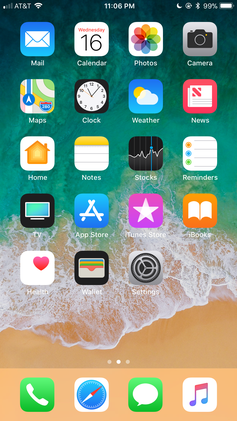This screenshot depicts a smartphone with a detailed beach-themed wallpaper. In the upper left-hand corner, the connectivity status shows one bar for AT&T, accompanied by a Wi-Fi icon. Centrally located at the top, the time is displayed as 11:06 p.m. Several small notification icons are visible to the right of the time, culminating in a battery icon in the upper right corner, which indicates a nearly full charge at 99%.

The background image of the screen showcases serene ocean water reaching up onto a sandy beach. The water's color transitions from a dark greenish-blue at the top to lighter shades as it approaches the shore, ultimately becoming white against the light brown sand, creating a calming gradient effect.

At the bottom of the screen, a tan-colored navigation bar features four essential icons: a phone, internet browser, green square for messaging, and a white square with two colorful musical notes denoting a media app. The main part of the screen is organized into five rows of app icons, neatly arranged for easy access.